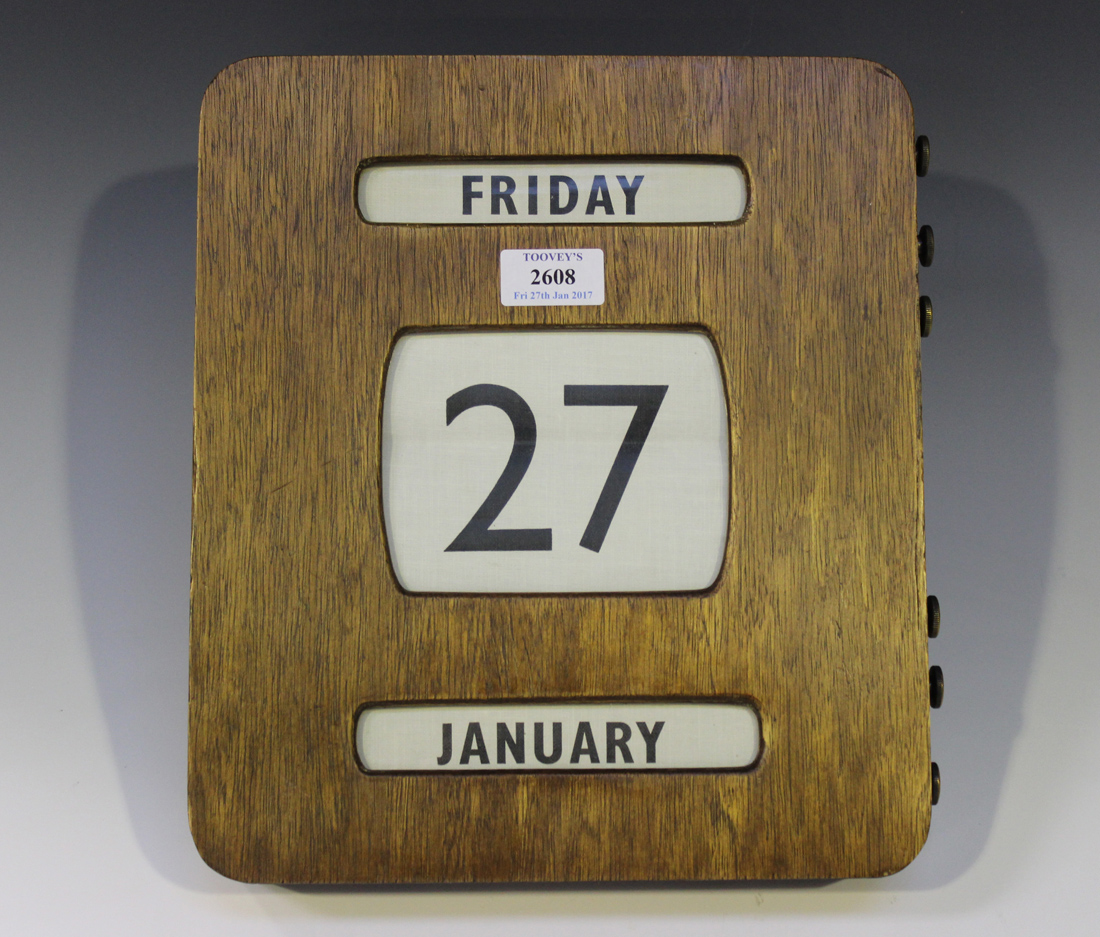The image depicts a vintage-style wooden calendar with a light gray background. The calendar is slightly rectangular, about six inches wide and five inches high. The wooden part has a honey brown color and features beveled edges. At the top center of the wood, there's an elongated oval with a light gray background and bold black text that reads "Friday." Beneath this, there's a small white rectangular sticker with the text "Tubbies 2608, Friday, 27th January 2017." Below the sticker, in the center of the wood, is a large square with beveled edges and a light gray background that prominently displays the number "27" in bold black print. At the bottom, another elongated oval with a light gray background and black text reads "January." On the right-hand side, there are three metallic knobs each on the top and bottom, which can be turned to change the date.